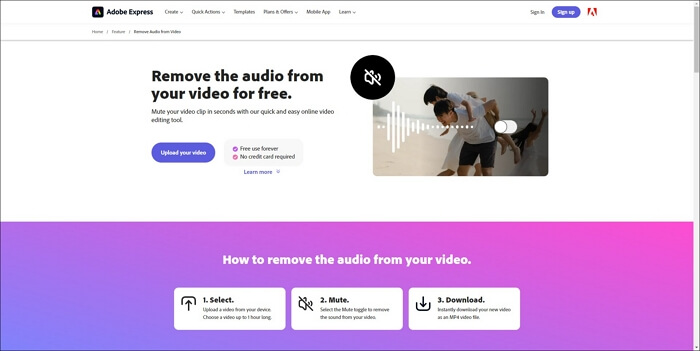**Detailed Caption:**

The image highlights a feature within the Adobe Express platform, which can be accessed through the app, software, or website. At the top left corner of the page, the "Adobe Express" logo is prominently displayed. The main focus of this page is a tool that allows users to remove audio from their videos for free, as indicated by the text, "Remove the audio from your video for free."

The page also provides a step-by-step guide on how to use this tool:

1. **Select your video:** Users begin by uploading the video from which they wish to remove the audio.
2. **Click on 'Mute':** Once the video is uploaded, users need to choose the mute option to remove the existing audio track.
3. **Download the video:** After muting, users can download the video. The downloaded file will no longer have any audio embedded in it.

With this feature, users can either post the video without any sound, ensuring that viewers cannot enable audio, or they can overlay the video with a new audio track to customize the content further. Thus, Adobe Express offers a straightforward and user-friendly solution for managing audio in video files.